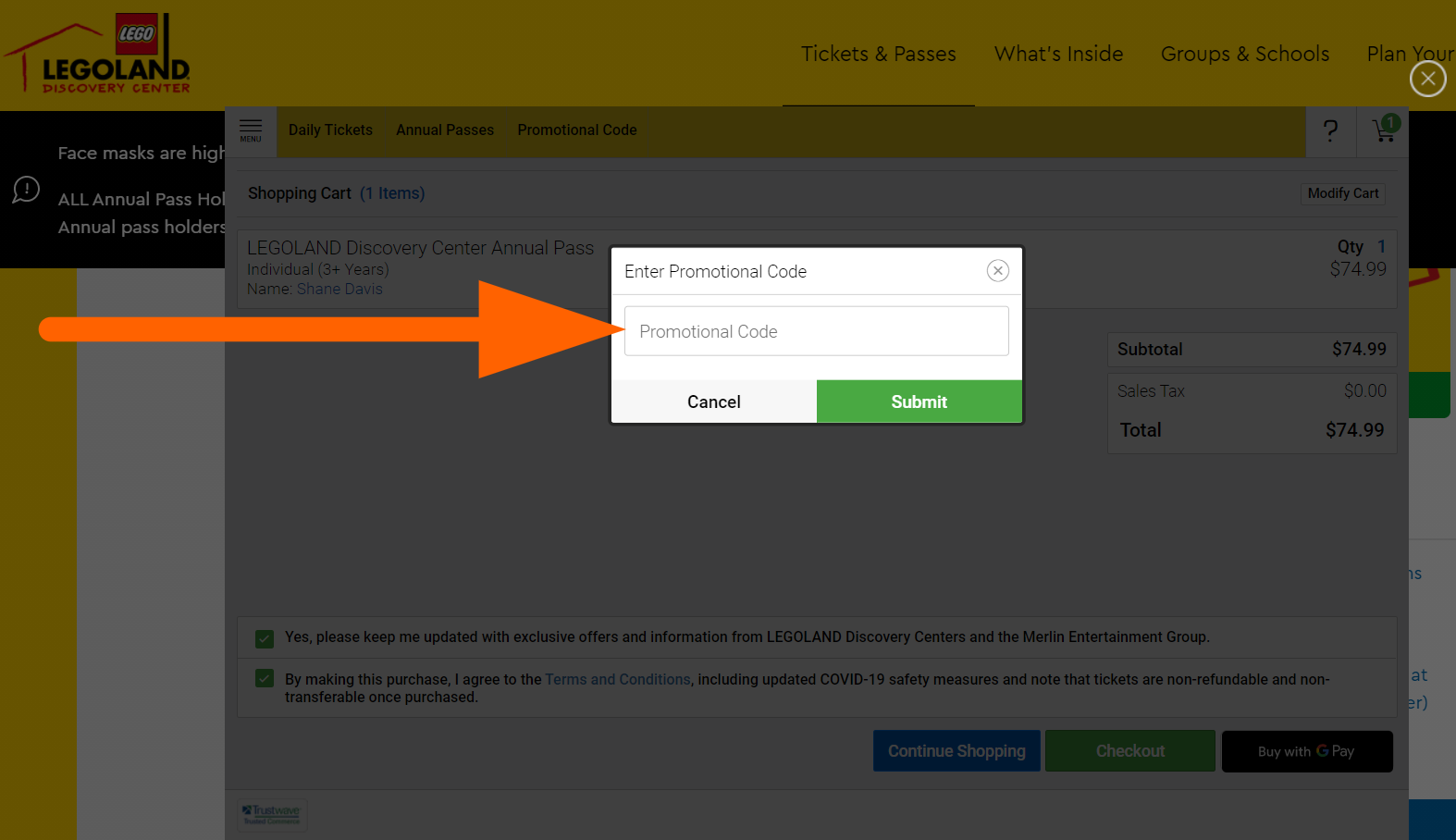The image showcases the Legoland Discovery Center website's layout. At the top of the screen, a prominent yellow bar spans the width, with a matching vertical yellow bar running down the left side. In the top left corner, there's a red outline of a building, featuring the iconic red Lego symbol with white lettering. Below the Lego logo, "Legoland" is displayed in black, and "Discovery Center" is written in red.

On the right side of the top bar, partially visible menu options include "Tickets & Passes," "What's Inside," "Groups & Schools," and "Plan Your..." The webpage underneath contains a black bar with various pieces of information set against a white background.

Centrally, a pop-up menu is present with options for daily tickets, annual passes, and a field for a promotional code. The shopping cart icon indicates it contains 1 item: a Legoland Discovery Center Annual Pass under the name Shane Davis, priced at $74.99. Additionally, another pop-up appears prompting users to enter a promotional code, if available, to receive a discount on the annual pass.